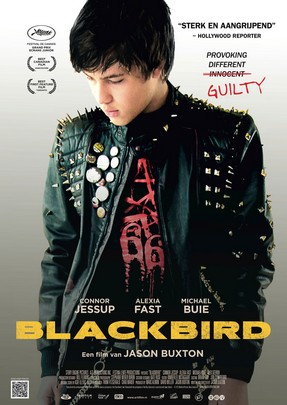The magazine cover features a young man with short black hair and bangs, looking down to his left. He wears a black leather jacket adorned with studs on the front and spikes on the shoulders, over a black and red t-shirt. At the bottom center of the image, the title "BLACKBIRD" is prominently displayed in large, all-caps yellow letters. Above the title are the names Connor Jessup, Alexia Fast, and Michael Buie in white text. To the upper right of his head, a quote reads, "Sturck on group hands. Hollywood Report provoking different," with the word "INNOCENT" dramatically slashed out in red and replaced with "GUILTY" in all-caps red letters. The lower left-hand corner contains a QR code and additional small white text that is unreadable. The phrase "Ein Film von Jason Buxton" is also visible, emphasizing the director's name. Overall, the cover suggests a gritty, provocative theme, with its dark color palette and striking visual elements.